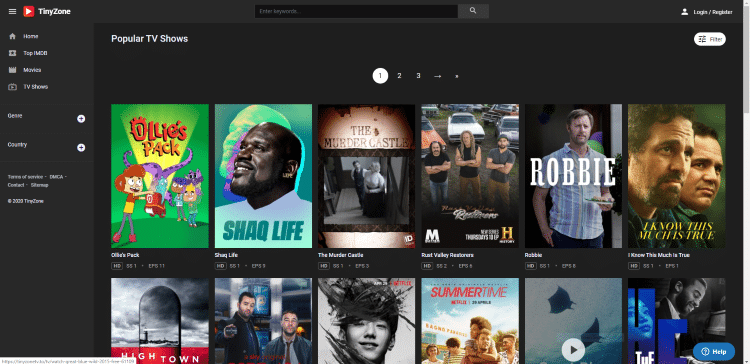The image depicts a dark-themed website interface with a predominantly black background. A slightly lighter shade of black outlines the top and left sides, forming a subtle border. At the top, there's a search bar with the placeholder text "enter keywords" in white font, accompanied by a white magnifying glass icon inside a small box to its right.

Adjacent to the search bar, three horizontal lines, often representing a menu, are stacked next to a red square containing a white triangle pointing to the right — likely a play button icon. Close to this is a small area with white text displaying the capital letters "T" and "Z."

Below these elements are navigation options labeled as Home, Top, I, M, C, O, Movies, TV Shows, and an illegible word followed by "Country." A white circle with a plus sign inside it is situated nearby. Further down, three numbers (1, 2, 3) appear inside white circles, arranged in a linear sequence.

The main content area showcases a selection of movies, divided into two rows: the upper row displays six movie options in full view, while the lower row appears partially visible, with the bottom half of the images cut off.